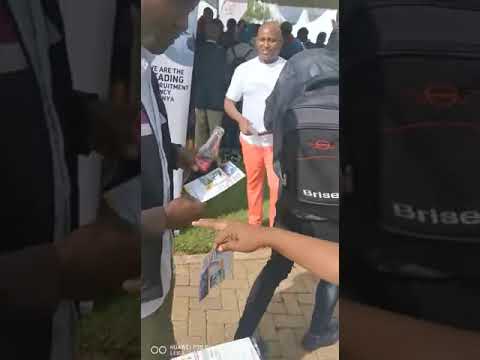In this detailed depiction of a social media video screenshot, possibly from Instagram or Facebook, the scene is set at an outdoor event, perhaps on a university campus. The ground beneath articulates a spatial division with a tan brick path extending from left to right, transitioning into a grassy expanse. Dominating the focal point is a bald black man, his head subtly illuminated by sunlight. He is attired in a white shirt and orange pants, holding an unspecified object around his waist with his right arm, his left hand out of view.

To his right, partially turned away from the camera, stands another man in a black jacket and jeans, a black backpack adorned with a logo at the top and white text below. This individual appears to be engaging with a pamphlet, indicative of the event's informational nature. To the left of the bald man, a third individual glances down at a pamphlet, holding a glass bottle of Coca-Cola in his left hand. He is dressed in a dark blue zip-up sweater with a white shirt underneath.

In the lower right foreground, the partially visible hand of another participant points towards the bald man, holding a pamphlet secured with a paper clip.

The converging energies and interactions depicted suggest an assembly aimed at disseminating information and rallying support, capturing the essence of community engagement.